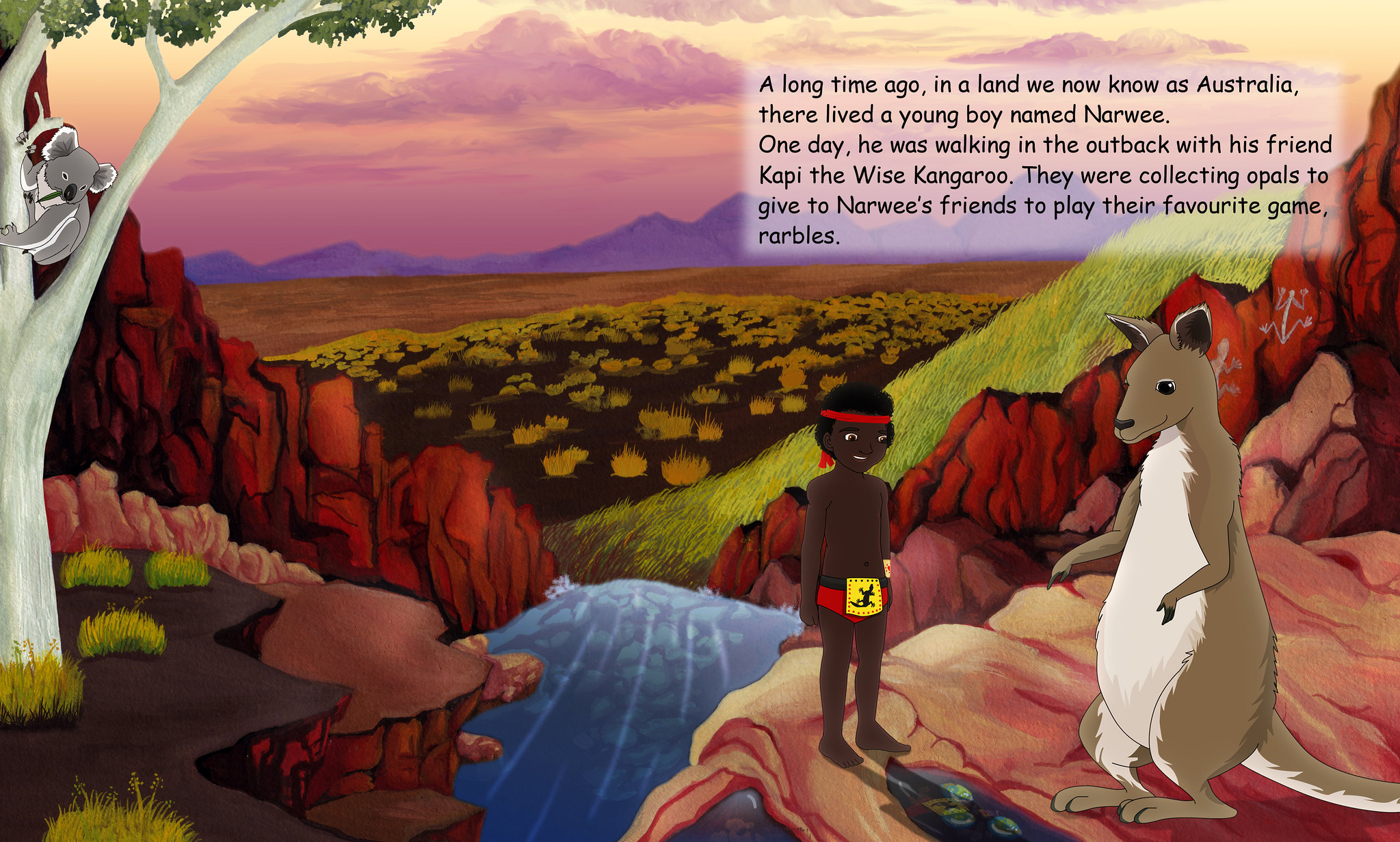This colorful rectangular illustration, likely from a children's book or a video game, presents a scene from the Australian outback. The viewer gazes down at an angle over a small, narrow waterfall or stream. On the left side, a rocky, steep shoreline ascends to a plateau where a tree stands, and a koala clings to one of its branches, looking down. Adjacent to the tree's peak rock formation, the right side features a flat area with a large kangaroo standing on its hind legs and an indigenous boy nearby. The boy, identified by his red bandana around his forehead and shorts, stands beside the kangaroo. The background slopes gently down into a meadow abundant with flowers, extending to a distant horizon marked by mountains, sky, and clouds.

A text bubble at the top reads: "A long time ago in a land we know as Australia, there lived a young boy named Narwee. One day he was walking in the outback with his friend Cappy the wise kangaroo. They were collecting opals to give to Narwee's friends to play their favorite game marbles." The image vividly evokes a sense of adventure and companionship in a vibrant, natural setting.